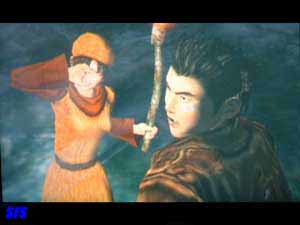The image appears to be a detailed, digital artwork, possibly a still from a video game or an anime, such as Shenmue. It features prominent black borders at the top and bottom of the screen with small, blurry blue writing on the bottom left, possibly indicating the letters "SFS." The focus is on two characters at the center of the scene. One character, a female, is depicted holding a stick with a flame at the end. She is dressed in an orange outfit with a matching light brown or orange beret, and a brown turtleneck or cowl neck underneath. Her sleeves are flared and loose, and she is seen covering her face with one hand. The other character, a male, is turned slightly away, displaying short, spiky black hair and an Asian appearance. He is wearing a brown, ornate suit or armor that includes a vest and shoulder or chest protection. He faces towards the side, adding a dynamic element to the composition. The background is a blend of dark green, light brown, and gray colors, creating a blurry and darker atmosphere.